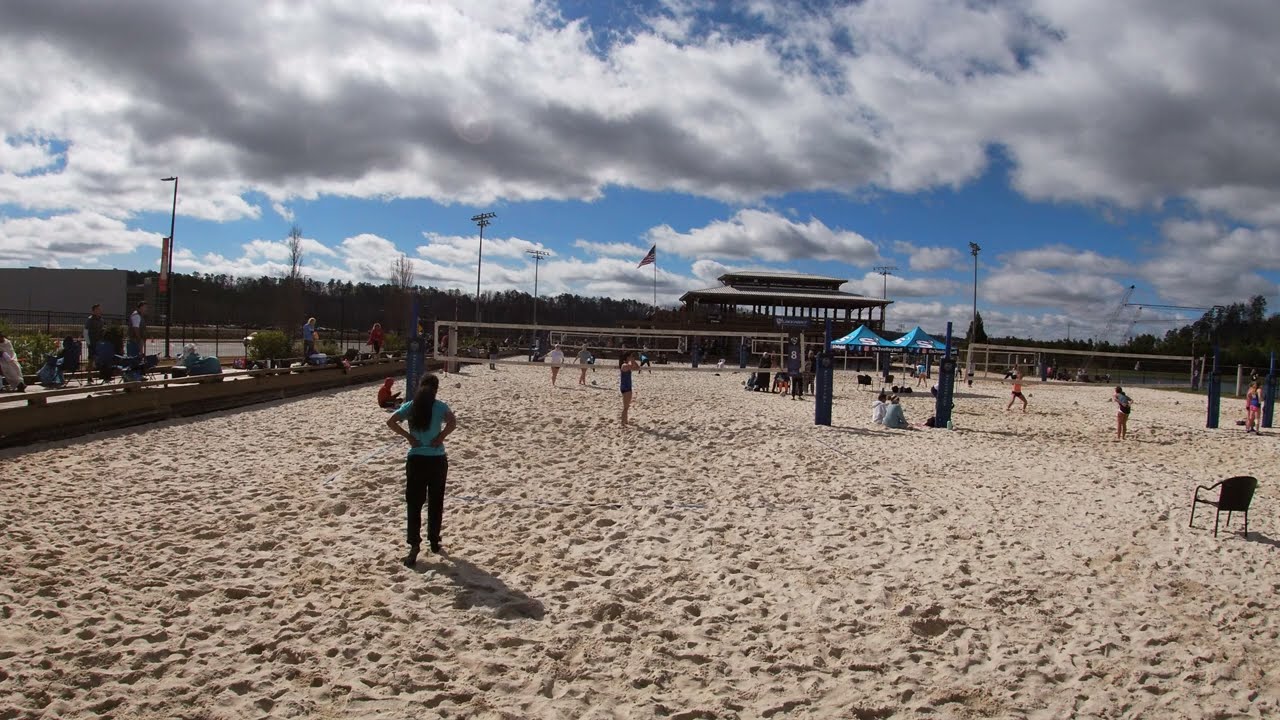The photograph captures a vibrant daytime scene on a sunlit beach volleyball area. Dominating the foreground is a woman with dark hair wearing a blue t-shirt and long pants, either playing or observing the game intently. She stands in front of a busy sandy area crisscrossed by a network of volleyball courts, bordered by a low cement divider. The sand, marked by numerous footprints, is testament to the many players engaging in various games across at least four nets, placed side-by-side. 

Around the courts, an array of colorful beach umbrellas, lawn chairs, and small blue-roofed tents are scattered along the right side and in the background, creating a festive atmosphere. Additional people can be seen lounging, seated or standing, observing the matches. Flats of umbrellas and simple structures punctuate the scene. On the beach to the left, onlookers gather behind a gray wall to watch the games, adding to the lively environment. 

Further back, towards the horizon, a pavilion-like building with dual roofs is visible, set against a backdrop of a treeline, with several light poles and an American flag on a flagpole standing out against the blue sky filled with fluffy white and gray clouds. This detailed tableau captures the essence of a bustling day at a beach volleyball event, blending the organized chaos of active play with the leisurely ambiance of beach life.